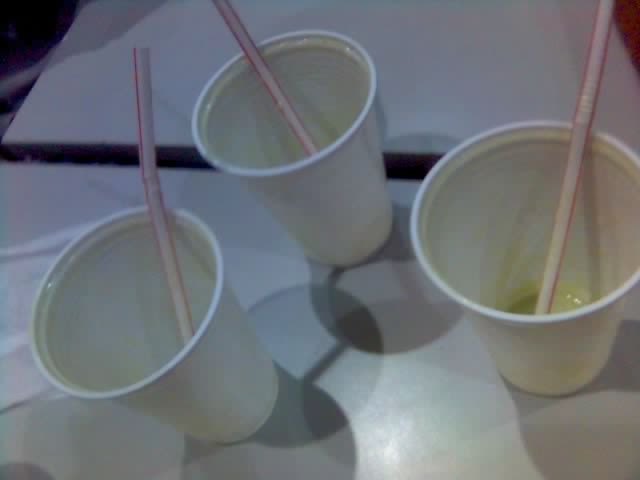The image depicts three small cream-colored disposable cups, each potentially holding 12 to 14 ounces, arranged in a triangular formation on a surface. Each cup is equipped with a white and red striped bendy straw. The cups appear empty except for some yellowish residue at the bottom and along the inside rim, suggesting they may have previously contained a lemon or vanilla milkshake. They are positioned on a white tabletop, which seems to have a dark line or gap, possibly indicating a seam between two sections of the surface. The cups are casting shadows, adding depth to the scene.